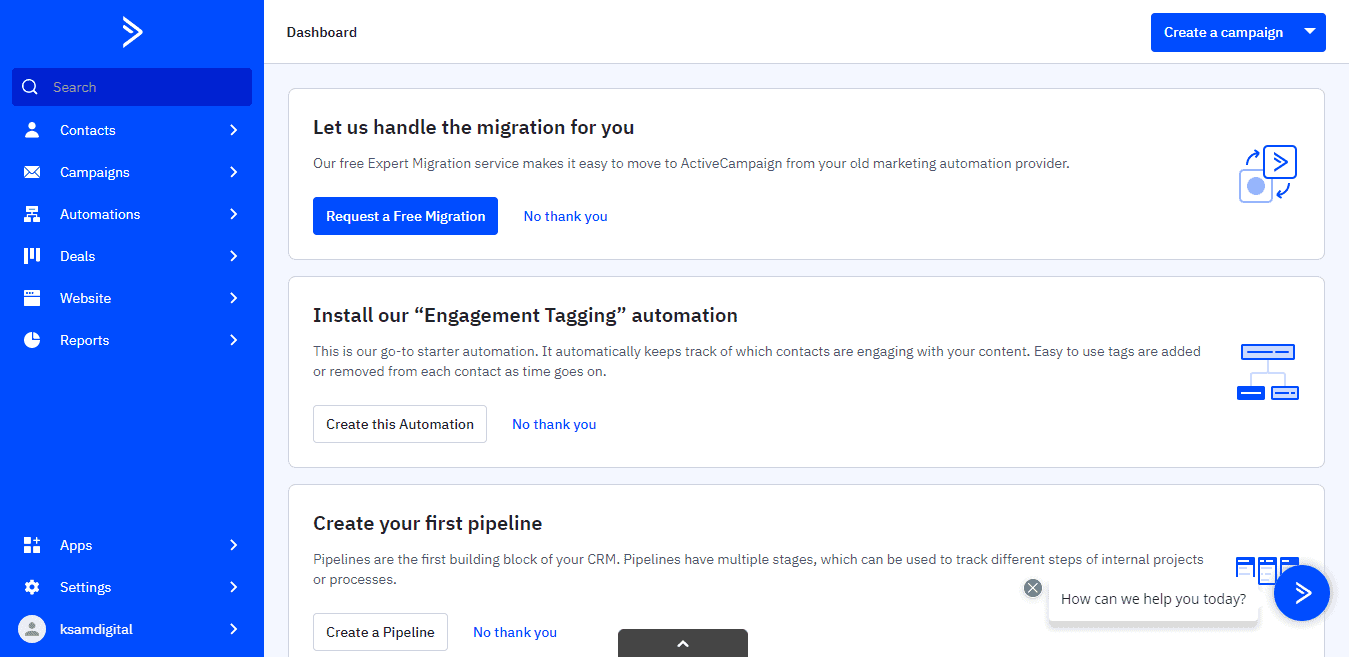This image is a screenshot of a computer application user interface. The interface features a bright blue sidebar on the left. At the top center of the sidebar is a white logo resembling a V rotated 90 degrees counterclockwise, with a shorter white line parallel to the top right leg of the V on the interior. Below this logo is a dark blue rectangle containing a white magnifying glass icon on the left and the light gray text “Search” to its right.

Underneath the search bar, there are rows of information organized in a structured format. Each row includes an icon on the left, followed by a couple of spaces, a label in white text, and a white arrow pointing to the right on the far right of the sidebar. The rows are as follows:

1. An icon of a computer monitor with two white squares underneath it, labeled “Automations”.
2. Three vertical white lines of different heights aligned to the top, labeled “Deals”.
3. A white webpage with a white header, labeled “Website”.
4. A white pie chart with the top right quadrant cut out, labeled “Reports”.

There is a considerable area of negative space below these rows, followed by three more entries at the bottom of the page:

1. A 2x2 grid of objects with three filled squares (top left, bottom left, bottom right) and a plus sign in the top right, labeled “Apps”.
2. A cog icon, labeled “Settings”.
3. A white circle containing a medium gray icon of a person, labeled “KSAM Digital”.